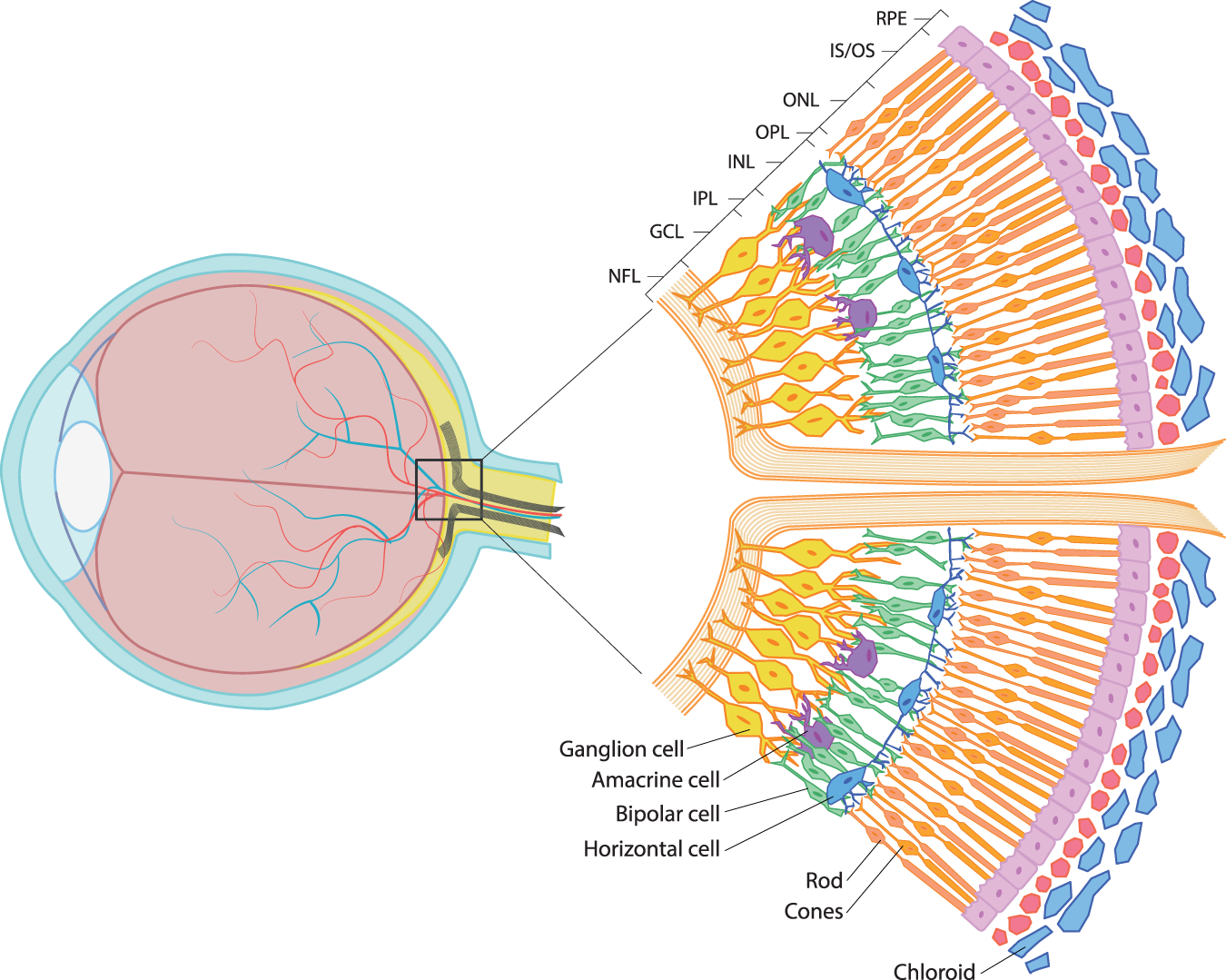This detailed illustration of the eye focuses on a magnified section of the back portion, showcasing the intricate layers and components involved in visual processing. On the left, a small depiction of the eyeball in blue and pink highlights the specific area being zoomed in on. To the right, the enlarged section intricately displays various labeled parts: the ganglion cell, amacrine cell, bipolar cell, horizontal cell, and rod and cone layers. Additionally, the schematic includes color-coded layers marked with acronyms like NFL (Nerve Fiber Layer), GCL (Ganglion Cell Layer), IPL (Inner Plexiform Layer), INL (Inner Nuclear Layer), OPL (Outer Plexiform Layer), ONL (Outer Nuclear Layer), ISOS (Inner and Outer Segments), and RPE (Retinal Pigment Epithelium). The outermost layers feature the choroid, depicted in blue. Overall, this comprehensive diagram combines descriptive labels and distinct color codes to elucidate the complex structure of the eyeball's posterior section.